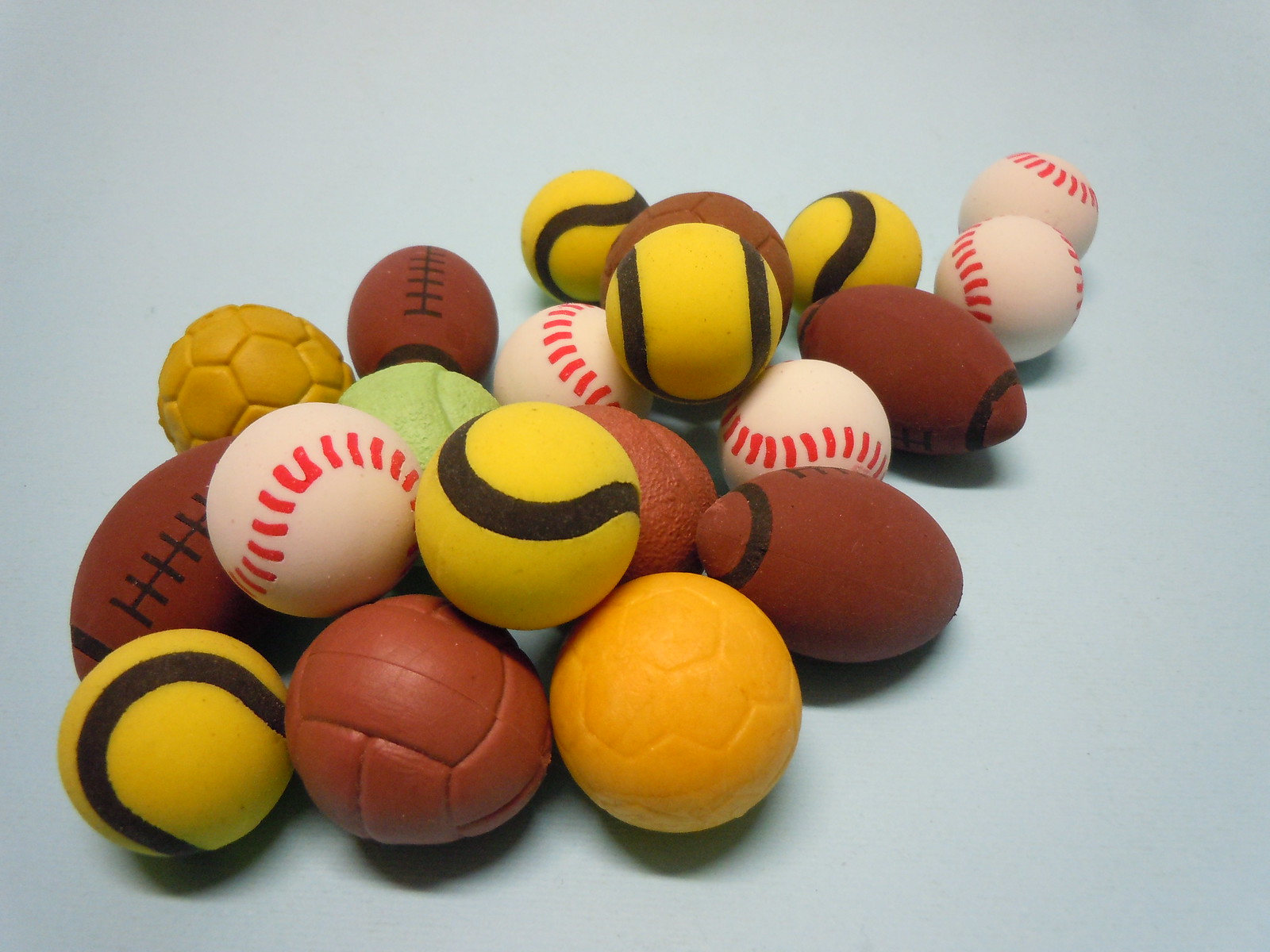The image depicts an artwork or a photograph featuring a collection of sports balls displayed on a light blue surface. There are approximately 15 to 20 balls, which include various types of sports balls such as baseballs, tennis balls, footballs, soccer balls, and volleyballs. The balls are distinctly detailed and made of a soft, plush material, resembling toys rather than functional sports equipment.

The baseballs are painted in white with either pink or red stitching, while the tennis balls are yellow with black markings. The footballs are brown with black laces, and there is a notable presence of multiple footballs. The soccer balls come in different designs, including solid yellow and orange variations. Additionally, there is a brown-colored ball that appears to be a volleyball.

All the balls are slightly larger than normal sports balls and are jumbled together in a pile. The material and construction suggest they are intended to resemble soft stuffed toys, suitable for children or pets. The repetitive appearance of certain balls, such as baseballs and footballs, adds to the overall playful and artistic arrangement of the scene.